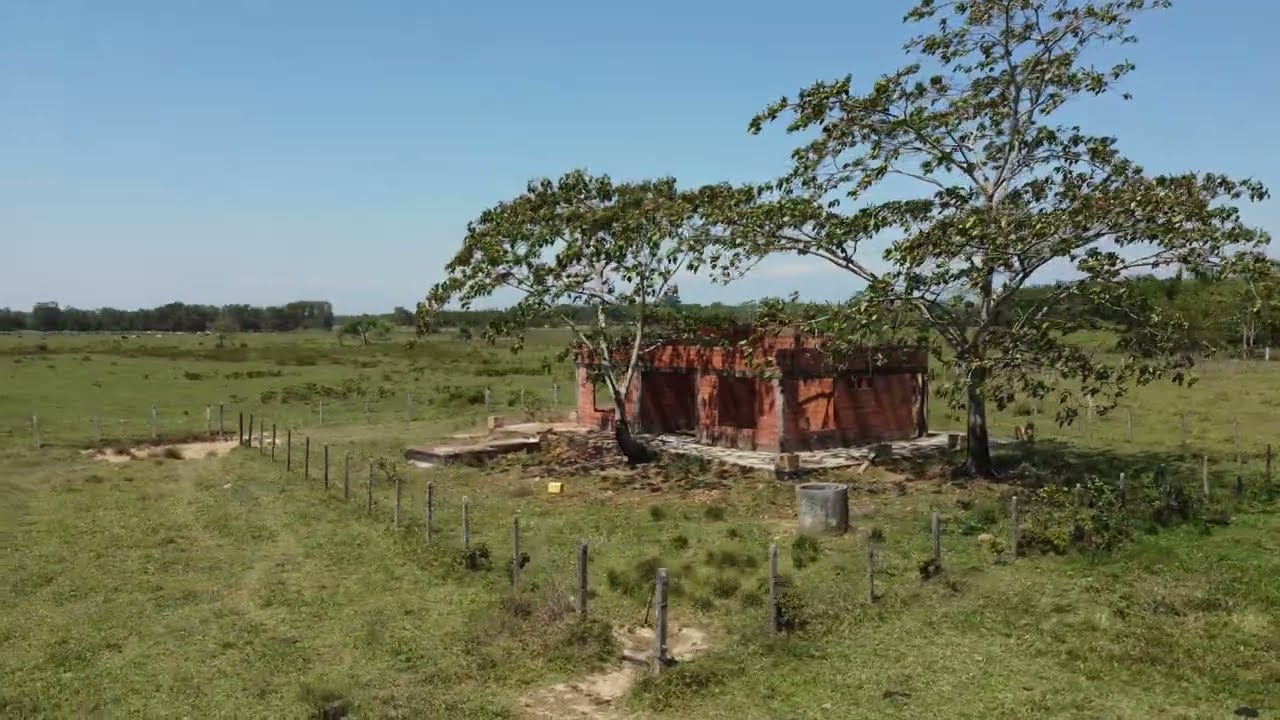This full-color outdoor photograph, taken during daytime, captures a horizontally rectangular scene dominated by a vast and open grassy field with some scattered bushes and clumps of taller grass. The backdrop of the image features a few distant trees and a bright, clear sky with a couple of faint clouds far in the distance. 

At the center of the photograph stands a small, dilapidated, red brick building on a concrete pad, which appears to be deserted and potentially abandoned. The building is flanked by two large trees that nearly obscure its roofline, which is flat and not distinctly visible. The windows and doorways of the building are just empty openings with no glass or doors, giving it a rundown appearance. The entire structure is encircled by a wooden fence, possibly reinforced with barbed wire, adding to the sense of neglect.

In the far background, hidden in the dense grove of trees, there are barely distinguishable black and white cows grazing. The absence of people or other animals in the immediate foreground and midground adds to the solitude of this deserted scene.